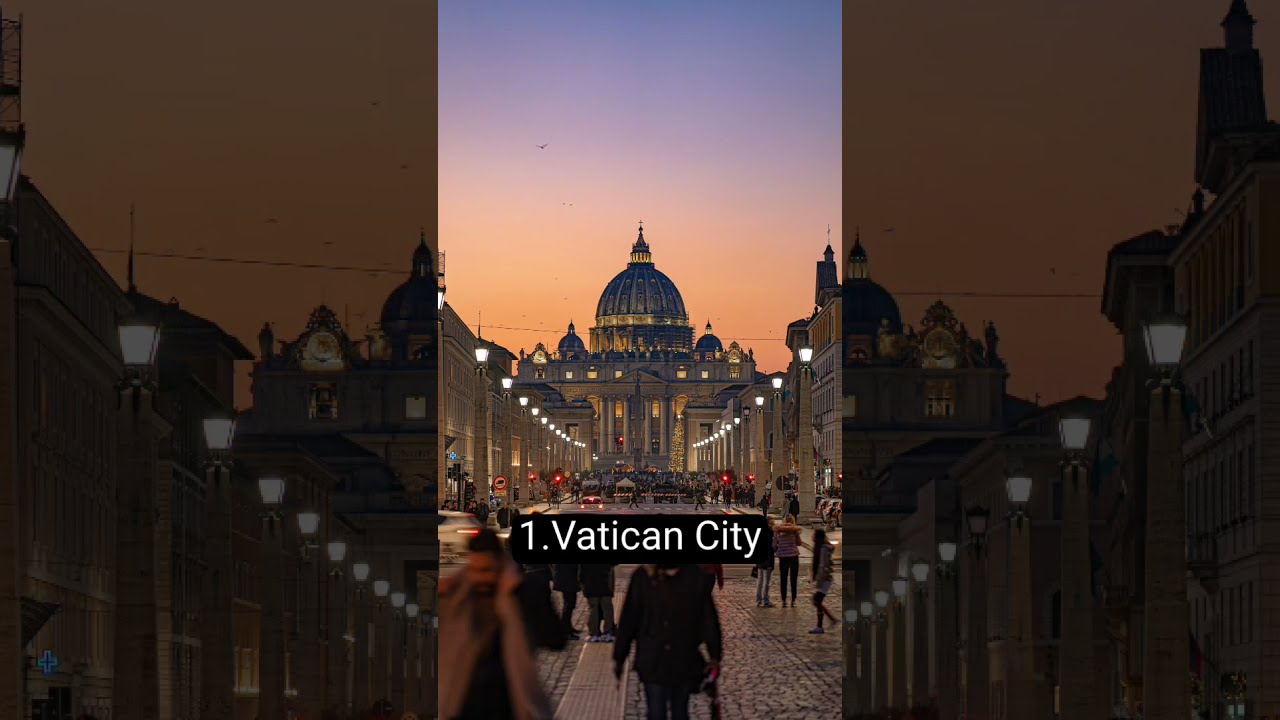This is a vertically oriented, color photograph capturing Vatican City at either sunrise or sunset, characterized by a gradient sky transitioning from a peach hue to a lilac lavender. The iconic dome of Saint Peter's Basilica stands prominently in the upper two-thirds of the image, flanked by stone buildings and framed by twin rows of lights. The lower third features a cobblestone plaza bustling with pedestrians, most with their backs turned, except for a blurred figure in the lower left corner. The entire scene is bordered by darkened bars, drawing attention to the warm hues and architectural grandeur. At the bottom, a black box with white lettering states "1. Vatican City," grounding the image in its historic location.